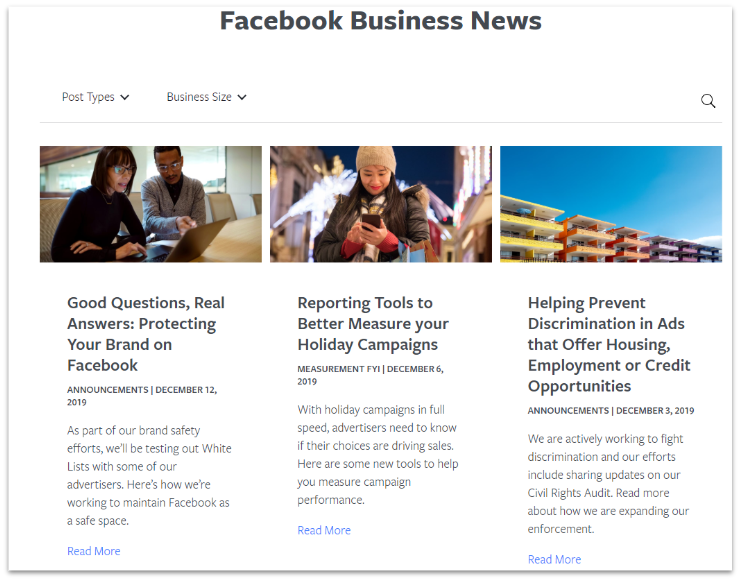The image is a screen capture of a webpage with a white background and the header "Facebook Business News" prominently displayed at the top in large black text. Below the header are three side-by-side photos accompanying feature articles.

The first photo on the left depicts a man and a woman seated side by side at a table, focused on a notebook computer in front of them. The caption beneath this image reads, "Good Questions, Real Answers: Protecting Your Brand on Facebook."

The second photo in the center shows a woman standing outdoors at night, with a black sky and rows of houses flanking her on both sides. She is engrossed in her smartphone. The caption beneath this image states, "Reporting Tools to Better Measure Your Holiday Campaigns."

The third photo on the right displays a clear blue sky with the upper stories of several tall buildings in view. The caption under this image reads, "Helping Prevent Discrimination in Ads that Offer Housing, Employment, or Credit Opportunities."

These images and captions collectively depict an informative webpage focused on providing business-related updates and tools for Facebook users.